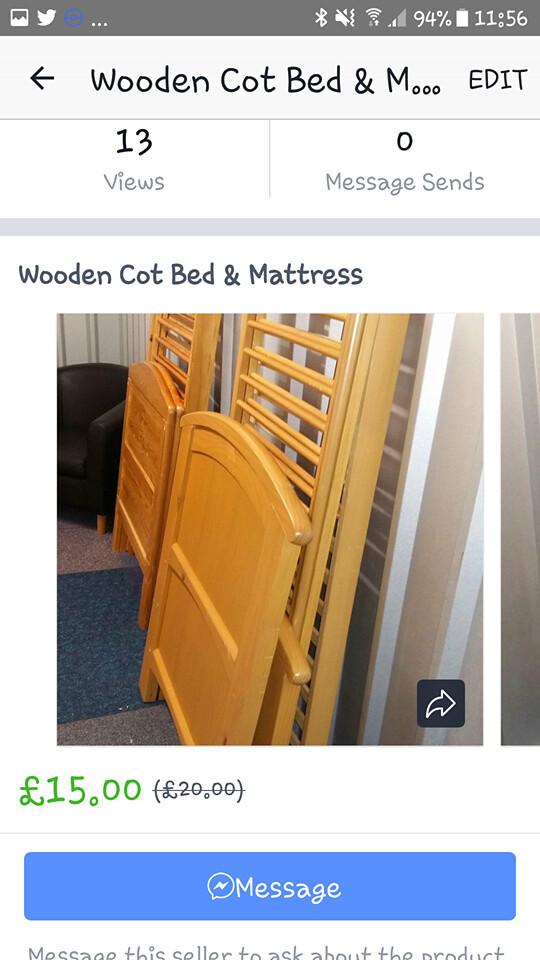The image is a screenshot, likely taken on an Android phone, displaying a Facebook Marketplace ad. The top section of the screenshot features a gray banner with icons: a TV, a white bird, and three dots, along with phone status indicators showing 94% battery and the time at 11:56. Below this, an arrow points left towards the text "wooden cot, bed, and m...edit." The ad details that the item is a "wooden cot, bed, and mattress," which has garnered 13 views but no messages sent. It features a picture of a wooden bed frame leaning against a white wall. The price is listed as 15 euros, reduced from 20 euros. Beneath the price, there is a blue button labeled "message," prompting potential buyers to contact the seller for more information about this single-sized bed, possibly designed for children.